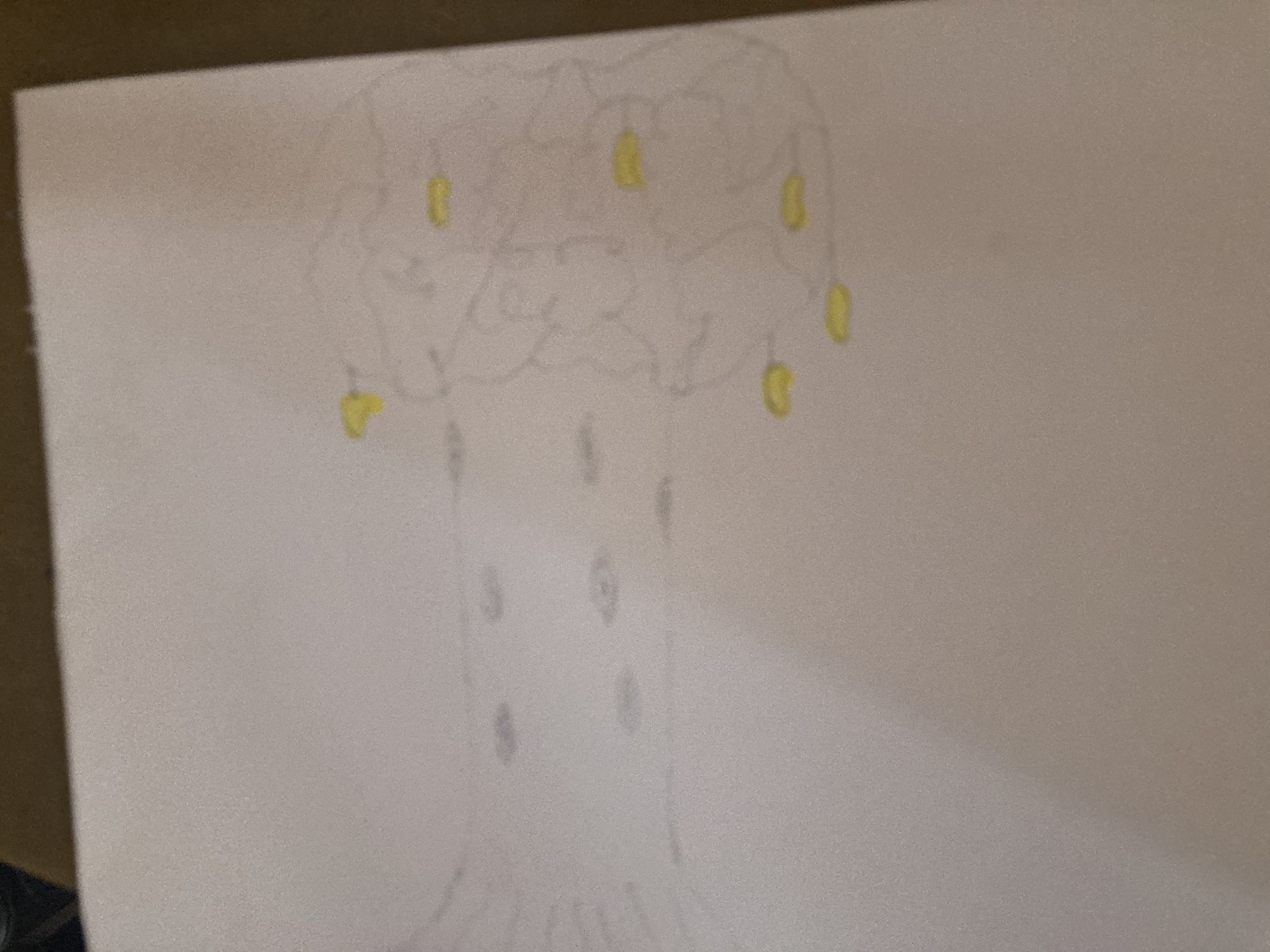In this blurry, poorly lit image, there is a white sheet of paper that is askew, set on a brown surface. The top left and bottom left corners reveal a light greenish background. The main focus of the drawing is a tree-like structure done in pencil. The tree features a round canopy with intricate swirls and lines. The canopy extends twice as wide as the trunk, which has seven black knots or spots and dark grey lineage descending. From the branches of the tree hang six yellow fruit—some describe them as leaves, others as yellow peppers—dangling symmetrically on either side. At the bottom of the tree, roots are faintly visible. The shadow cast across part of the paper and the angle it's placed add to the overall sense of poor lighting in the image.